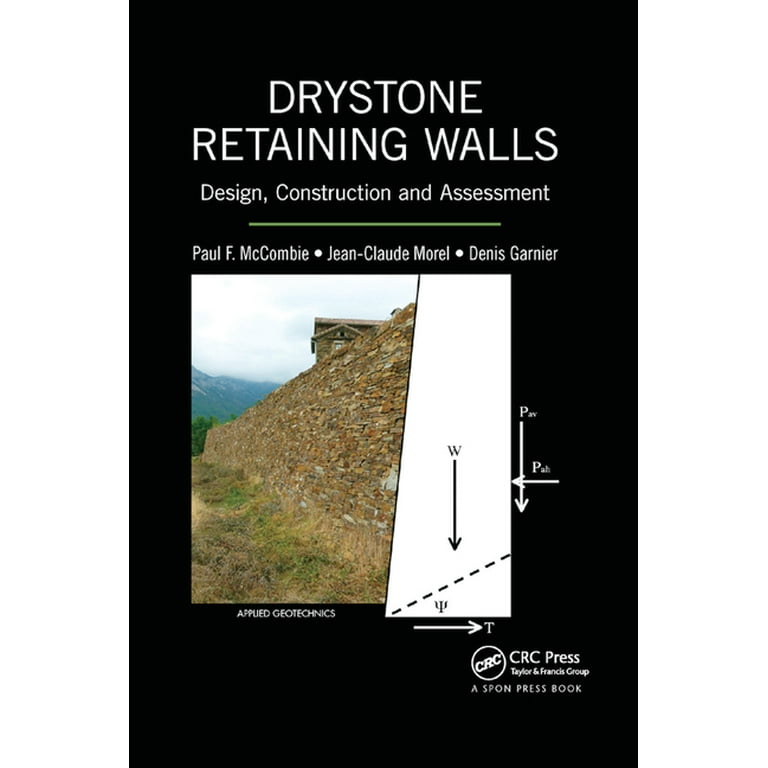The cover of the book titled "Dry Stone Retaining Walls: Design, Construction, and Assessment" is depicted against a black backdrop with prominent white text. At the top, the title is displayed in bold letters, and a thin green divider line separates it from the subtitle. The book features authors Paul F. McCombie, Jean-Claude Morel, and Denis Garnier. A large, centered color photograph illustrates a stone retaining wall supporting a house situated on a mountainous hillside under a cloudy sky. Next to the photograph is an architectural diagram with directional arrows labeled "W," "T," and "P." In the bottom right corner, the logo for CRC Press, part of the Taylor & Francis Group, is visible, along with the label "A Spon Press Book."